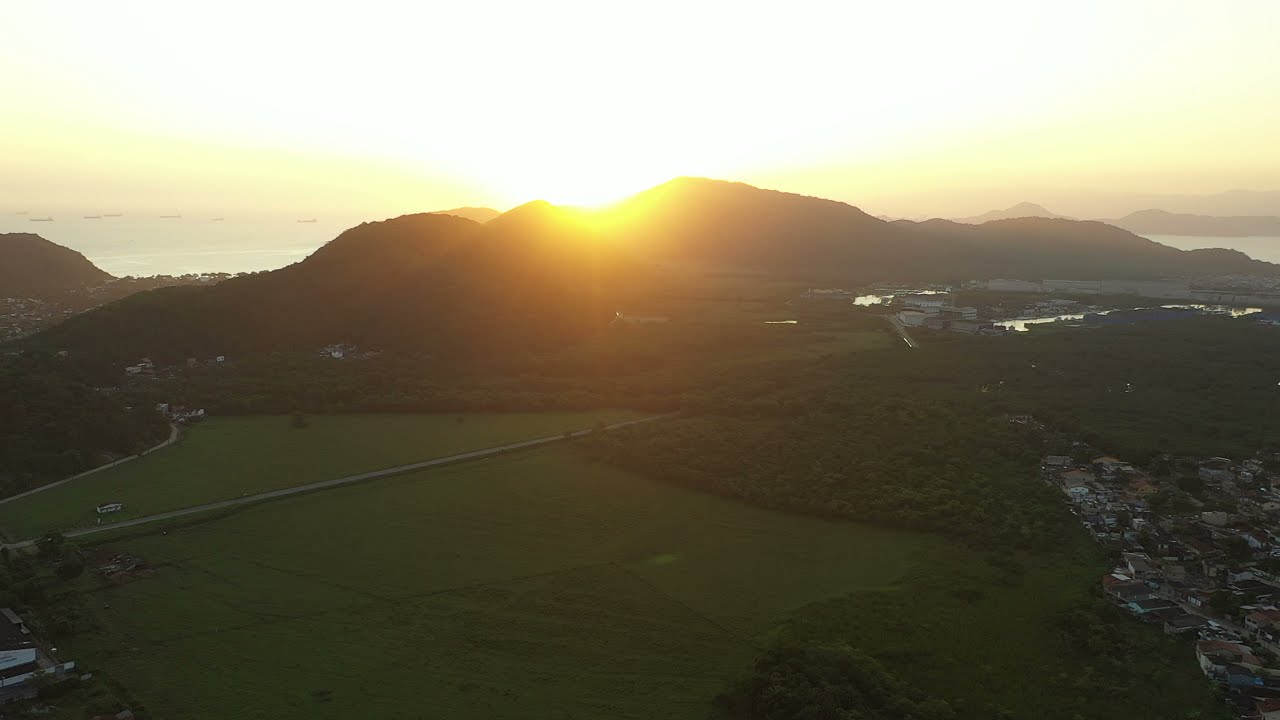This aerial photograph, taken from a drone or plane at elevation, captures a breathtaking scene of a sunrise or sunset over a vast, green field that stretches towards the bottom of the image. In the foreground, the bottom left corner showcases lush greenery, while the bottom right corner reveals a residential area. At the center of the image, running diagonally, a narrow road cuts through, leading towards the distant hills.

The hills themselves, possibly a series of them rather than a single peak, span the width of the image just below the center. The sun's brightness obscures much of the detail, casting a yellow hue over the terrain and creating a blend of bright white and warm tones of yellow and orange. In the background, a large body of water, which could be a lake, makes a subtle appearance near the edge of the hills. The vegetation near the residential area appears more like trees, though they look like shrubs from this height.

Overall, the photograph offers a sweeping view of the edge of a town, showcasing the interplay of natural and man-made elements illuminated beautifully by the sun rising or setting behind the hills, near a serene body of water.